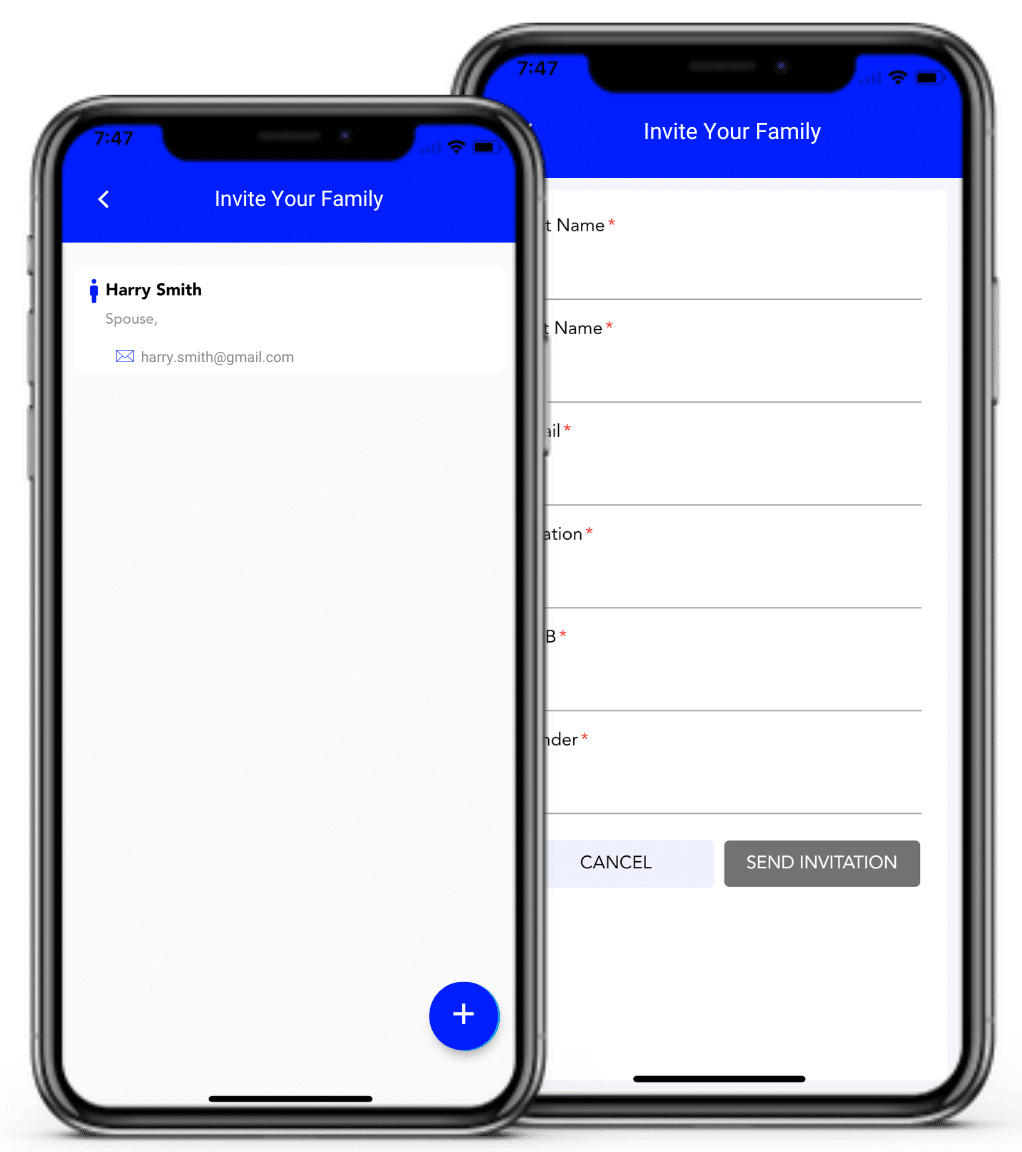This image features a detailed screenshot of a mobile application designed for inviting family members to join a specific platform or service. The screenshot is divided into two sections, each showcasing a different step in the invitation process.

On the left side, a smaller phone screen displays a user interface titled "Invite Your Family" at the top. Below this, the name "Harry Smith" appears with a label indicating "spouse," suggesting that the app automatically recognizes family relationships based on existing profile information. Users likely have the option to click on this profile to send an invitation directly to "Harry Smith" to join the app or website.

On the right side, a slightly larger phone screen offers a manual input form for inviting additional family members. This screen includes fields labeled "First Name" and "Last Name," alongside further fields for providing additional information such as email addresses and the invitee's relationship to the user. This manual entry method allows users to input necessary details to invite other family members not automatically recognized by the app.

Overall, the screenshot illustrates a user-friendly application interface aimed at simplifying the process of involving one's family in the app's ecosystem, either through automatic recognition of existing profiles or manual data entry.